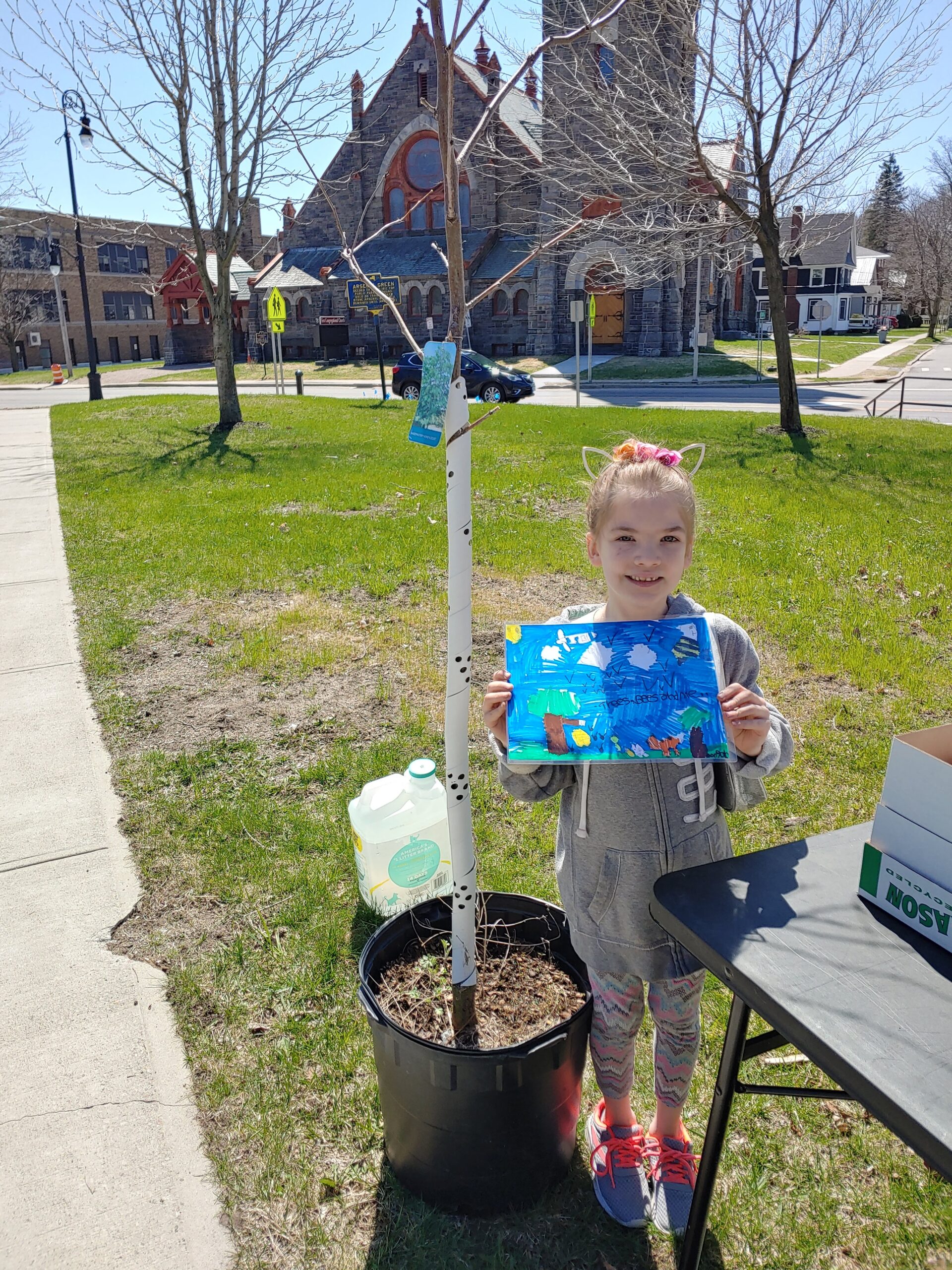In an outdoor scene resembling a small park or town center, a young girl, around eight years old, stands proudly holding up her watercolor painting that depicts an outdoor scene with trees, a blue sky, and clouds. The girl has blonde hair tied back and wears a headband with little cat ears adorned with pink flowers in the center. She is dressed in a gray oversized zip-up sweatshirt with "SC" on it, multicolored leggings in shades of red, purple, green, and blue, and lavender running shoes with bright pink laces. To her right is a small black folding table with a white box on it, set up on the grass. She stands next to a small tree planted in a black five-gallon bucket. The background features a stone gray church and a three-level brownstone building, hinting at a peaceful, community outdoor setting under a clear blue sky.